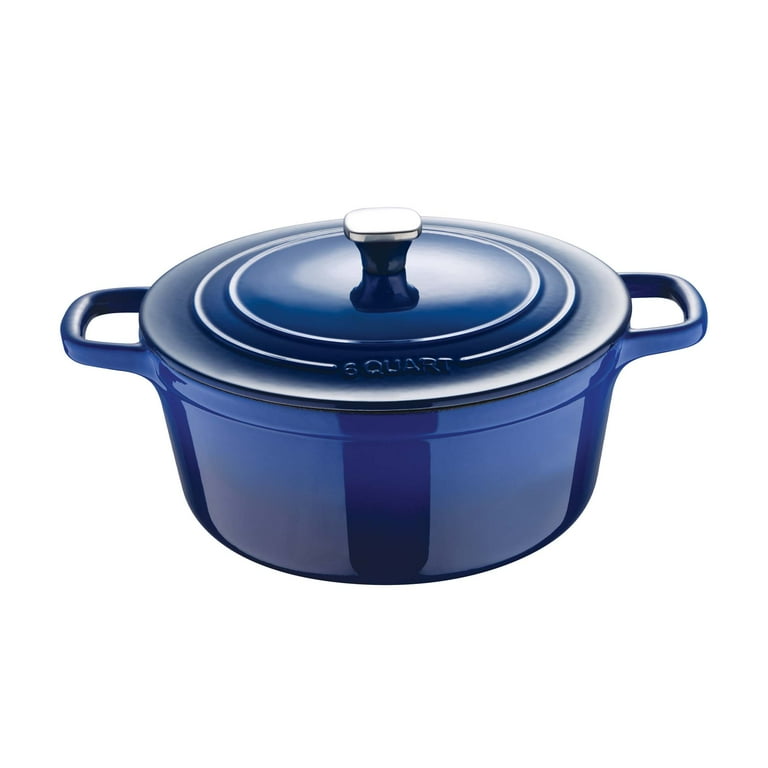This image features a dark blue, six-quart cast-iron Dutch oven, coated with ceramic and polished to a shiny finish. The Dutch oven sits centered against a stark white background, which accentuates its rich, deep blue color. It has two side handles, designed in a distinctive C-shape, and a lid adorned with a square knob that's rounded at the corners and silver in color. The lid also features two concentric circles around the knob. Although the brand name imprinted on the lid appears to spell something like "C-O-U-A-R-T," it is illegible. The outermost circle on the lid bears the inscription "six quart." The Dutch oven gleams under the light, showcasing a gradient effect from a darker blue at the base that gradually lightens towards the top.